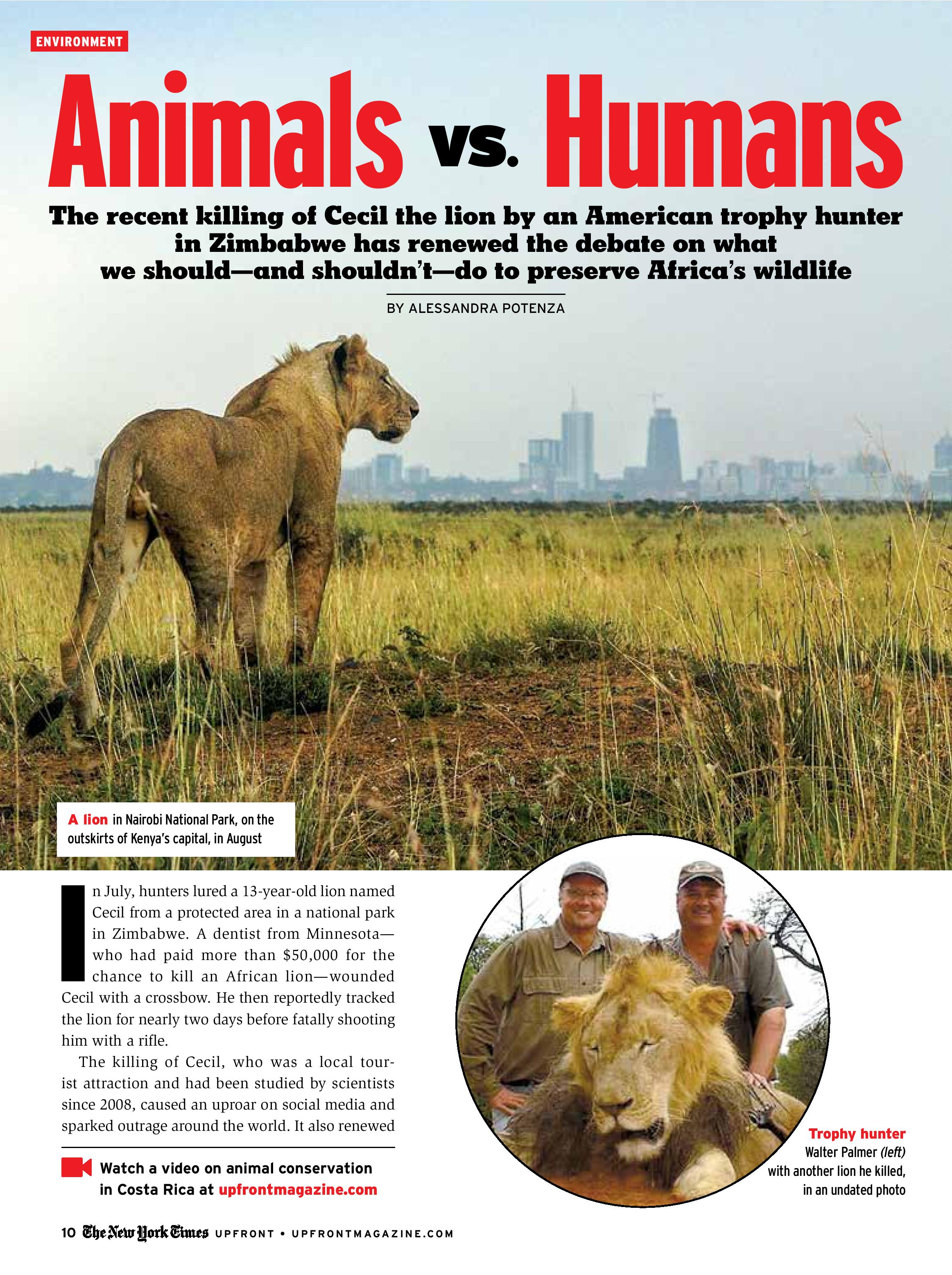**Detailed Caption:**

This image is a vertical screenshot of an article from The New York Times Upfront, found on upfrontmagazine.com. Dominating the top of the screenshot is a square photograph featuring a majestic lion known as Cecil. The lion, standing with his back to the viewer, is situated in a field of long grass and dirt, with a distant cityscape visible in the background. At the bottom of this photograph, a white text bubble highlights key information about the image.

The headline of the article, "Animals vs. Humans," is prominently displayed beneath the photograph. The article discusses the renewed debate around wildlife preservation in Africa, sparked by the controversial killing of Cecil the lion by American trophy hunter Walter Palmer. The article is authored by Alessandra Potenza.

Below this headline is a circular inset photo of Walter Palmer and another man standing with a different lion, also killed by Palmer, as noted by the accompanying black text to the right. The text reads, "Trophy hunter Walter Palmer (left) with another lion he killed in an undated photo," making it clear that this lion is not Cecil.

In the lower-left corner of the screenshot, the reader can find the page number "Page 10" and the publication details "The New York Times Upfront," along with the website URL "upfrontmagazine.com."